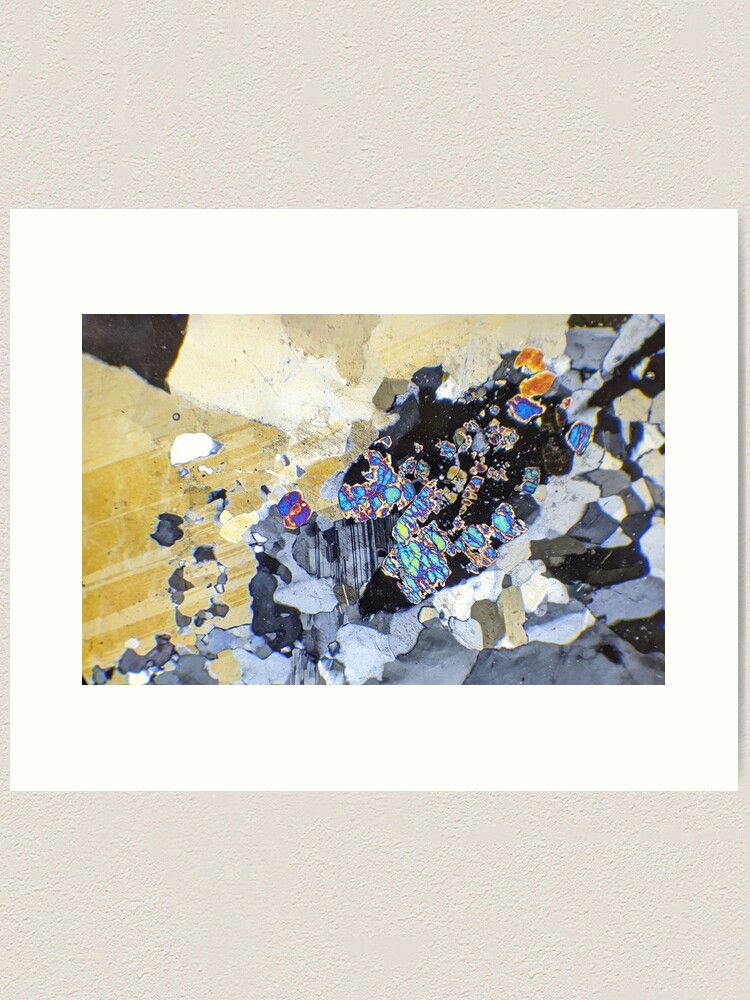The image features an abstract painting framed by distinct layers. The outermost border is light beige, with large, solid strips on the top and bottom. Inside this border is a white inner frame that encloses the painting. The painting itself is landscape-oriented and divided into two primary sections, separated by a diagonal line running from the bottom left to the top right. The left section features a mustard yellow-tan color, while the right section contains an array of light gray, dark gray, light blue, dark blue, and grey shapes scattered sporadically. The painting includes dark gray and black stone-like textures, adorned with colored bits in shades of purple, light blue, and white. There is also a noticeable golden-yellow, dusty floorboard-like texture at the bottom. Additionally, some light is reflecting in a manner that suggests the presence of a signature in the middle of the image.